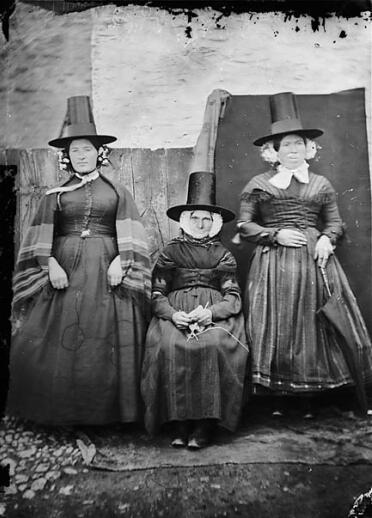This is a detailed black and white photograph from the 1800s or very early 1900s, depicting three women dressed in somber, high-collared, long-sleeved dresses that reach down to their feet, obscuring their legs but revealing their shoes at the very bottom. All three women are adorned with tall, stovepipe top hats that have wide brims. The woman in the center, who appears older and is seated, holds knitting needles and yarn, suggesting an air of domesticity and tradition. Flanking her are two other women, standing closely on either side, with the woman on the left draped in a striped shawl that stands out even in the black-and-white format of the photo. The backdrop appears to be a fence made of wood blocks, adding a rustic element to the scene. All three women wear solemn expressions, contributing to the overall austere and antiquated feel of the portrait.